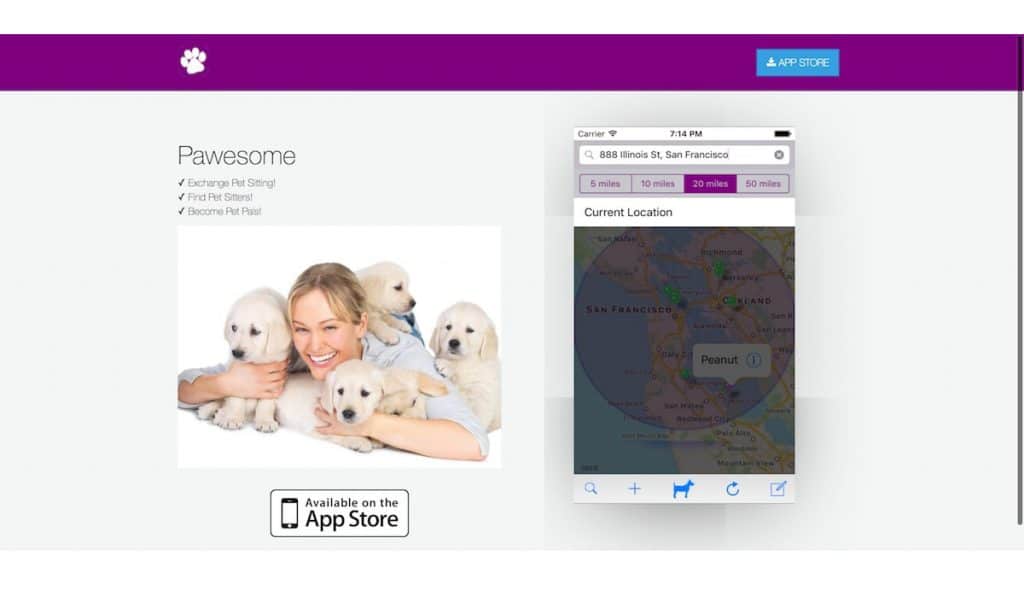This is a screenshot of an advertisement for a pet-sitting app named "Pawsome." In the center, there are two prominent images. On the left, a joyful woman is surrounded by four playful white puppies. She is smiling broadly, possibly laughing, with her arms lovingly wrapped around two of the puppies, while the other two endearing puppies clamber over her back and shoulder. Above this heartwarming scene, bold text reads "Pawsome." Beneath this title are three bullet points that outline the app's features: "Exchange Pet Sitting," "Find Pet Sitters," and a partially obscured "Become Pet" (the exact wording is difficult to read).

Beneath the image of the woman and her puppies, a logo indicates that the app is "Available on the App Store."

To the right is a screenshot of the app interface. It features a grayed-out map, likely where users can input an address to search for nearby services. A plum-colored banner across the top of this image includes a white paw print on the left and an "App Store" button on the right, complete with an icon suggesting a link to the App Store.